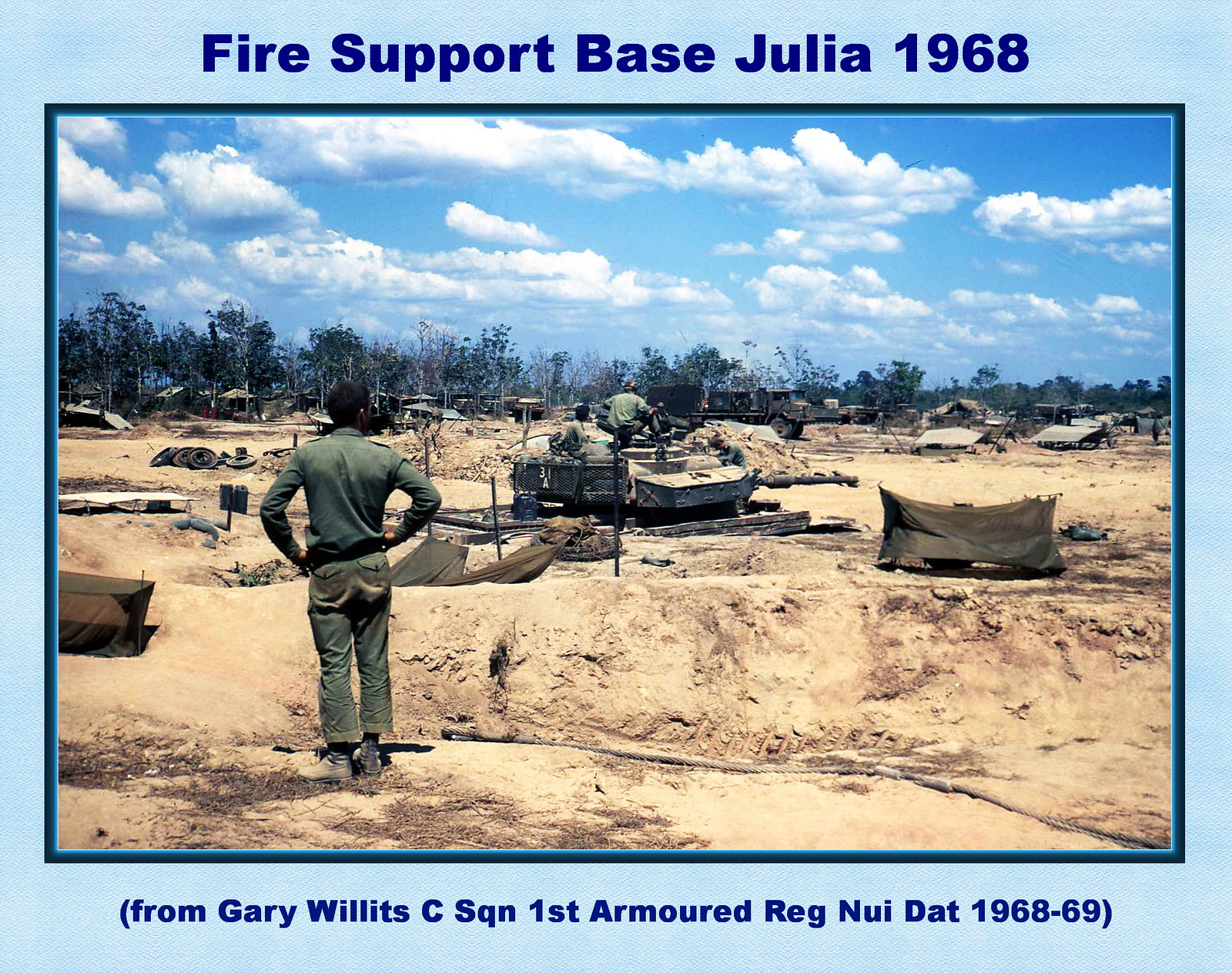This photographic image, encircled by a blue border, captures Fire Support Base Julia in 1968 during the Vietnam War. Set against a backdrop of a blue sky dotted with clouds, the scene depicts a barren sandy area with sparse vegetation, scattered trees in the distance, and ditches and foxholes throughout. Central to the composition is an armored vehicle, possibly a tank equipped with a machine gun, parked in a ditch or hole. Around it, a variety of tents—small individual pup tents and larger ones—are visible alongside berms of dirt. In the background, small buildings are dotted along the tree line.

In the foreground, a GI in olive green military uniform with his hands on his hips surveys the area. Another notable detail is a young black man, potentially an Australian, sitting on the tank and looking out towards the distance. At the bottom of the image, a caption reads: "From Gary Willitt’s C-Squadron, 1st Armored Regiment, 1968-69," clearly dating the photograph to the height of the Vietnam War.